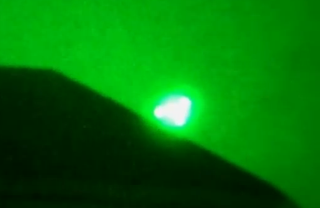The image is a night-vision photograph dominated by shades of black and green, with highly contrasting elements. An unidentifiable dark structure, possibly a hill or mountain, descends diagonally from the top left corner to just before the bottom right corner. Emerging from the midpoint of this slope is a strikingly bright, cone-shaped light with a halo effect, adding a mystical touch to the scene. The background features a light green sky, creating a distinct separation between the shadowed area and the illuminated parts. Despite its graininess, the photo's unique composition and stark color contrast make it visually compelling, though the exact nature of the depicted objects remains unclear.